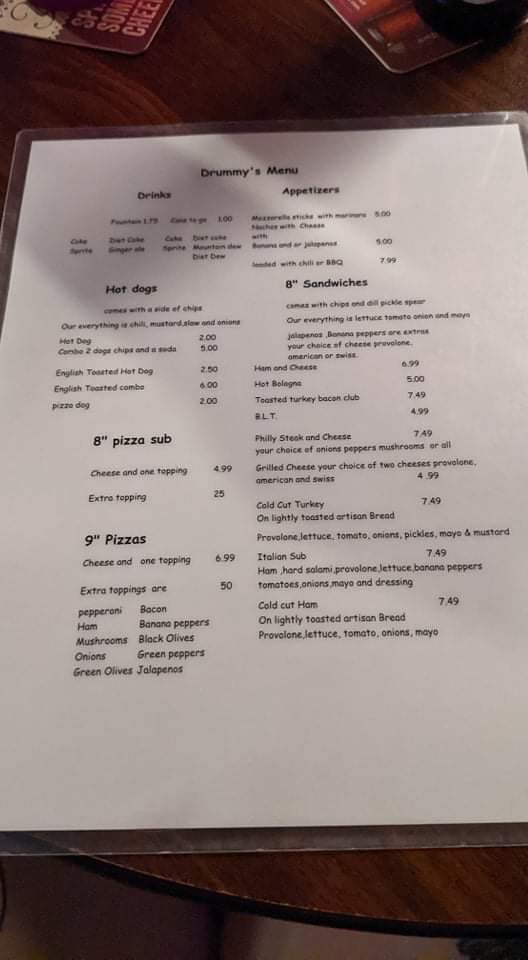The image showcases a laminated menu titled "Drummy's Menu" placed on a round table with a wood finish. The table, constructed from particle board with a laminate surface, shows signs of wear with visible scratches. The menu, printed on standard printer paper and laminated, features the text in the recognizable Comic Sans font. Categories listed on the menu include drinks, appetizers, hot dogs, 8-inch sandwiches, 8-inch pizza subs, and 9-inch pizzas. The menu is devoid of any photos or graphics, presenting a straightforward list of items. In the background, the edges of a couple of coasters peek out, hinting at drinks on the table, though only the shadows of the glasses are visible, suggesting the setting is a casual restaurant.